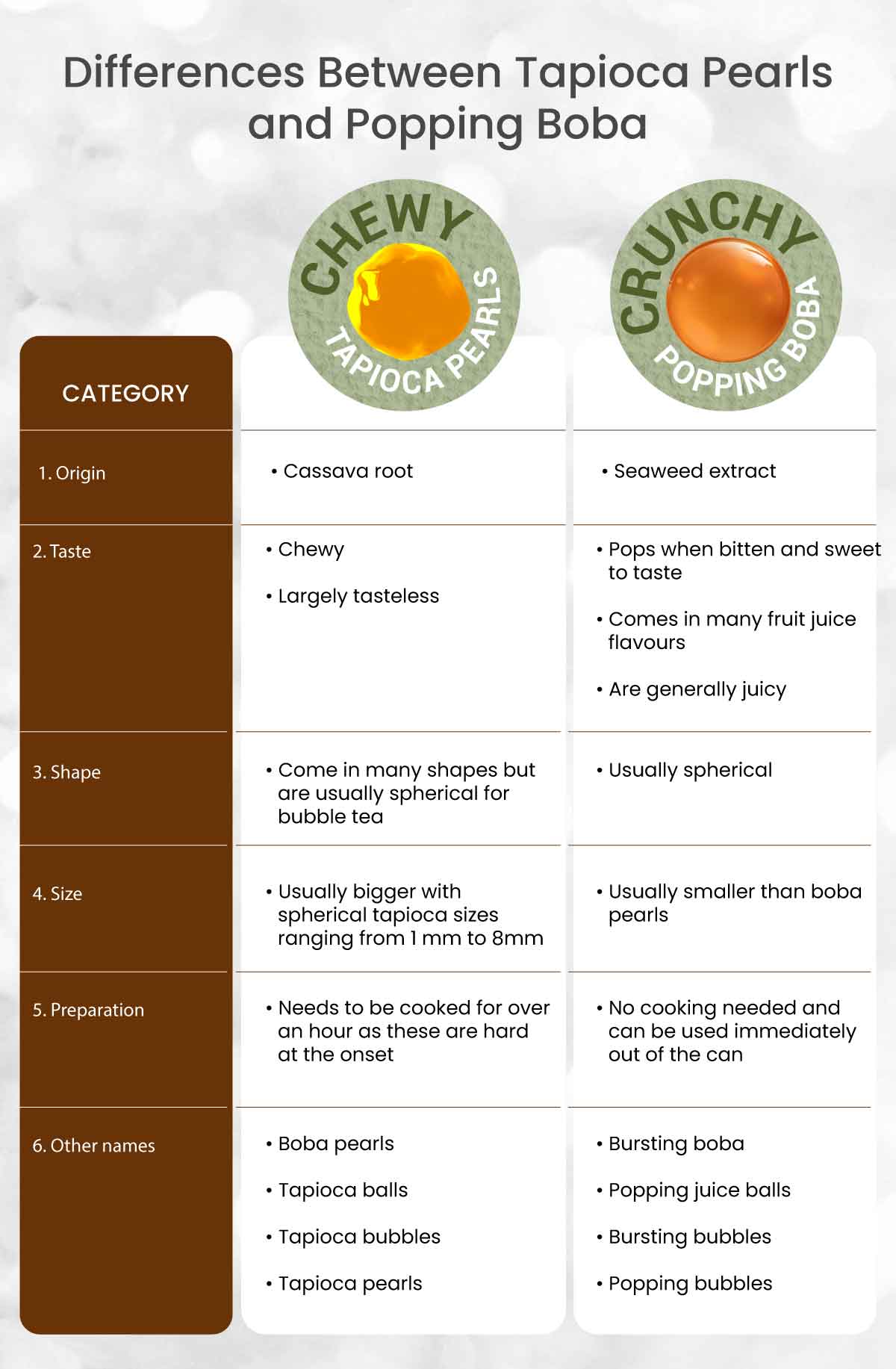The image is a detailed and vertically-oriented chart, set against a white background, with the heading "Differences between Tapioca Pearls and Popping Boba" at the top in black letters. The left section of the chart is dedicated to "Chewy Tapioca Pearls," and the right section to "Crunchy Popping Boba." Both sections provide various details about the respective items under the same categories: Origin, Taste, Shape, Size, Preparation, and Other Names.

In the "Tapioca Pearls" section, the origin is listed as cassava root and their taste is described as largely tasteless. They are usually spherical in shape, with sizes ranging from 1mm to 8mm, and require cooking for over an hour due to their hardness. They are also known by other names such as boba pearls, tapioca balls, tapioca bubbles, and tapioca pearls.

In the "Popping Boba" section, the origin is noted as seaweed extract. These pearls pop when bitten and are sweet to taste, often coming in various fruit juice flavors. They are generally smaller than tapioca pearls and also spherical in shape. Unlike tapioca pearls, popping boba requires no cooking and can be used straight out of the can. Other names for popping boba include bursting boba, popping juice balls, bursting bubbles, and popping bubbles.

Illustrations include a circle labeled "chewy" with an orange orb underneath for tapioca pearls, and a circle labeled "crunchy" with a similar orange orb for popping boba. The chart is organized with a brown rectangle on the left side detailing the categories sequentially.